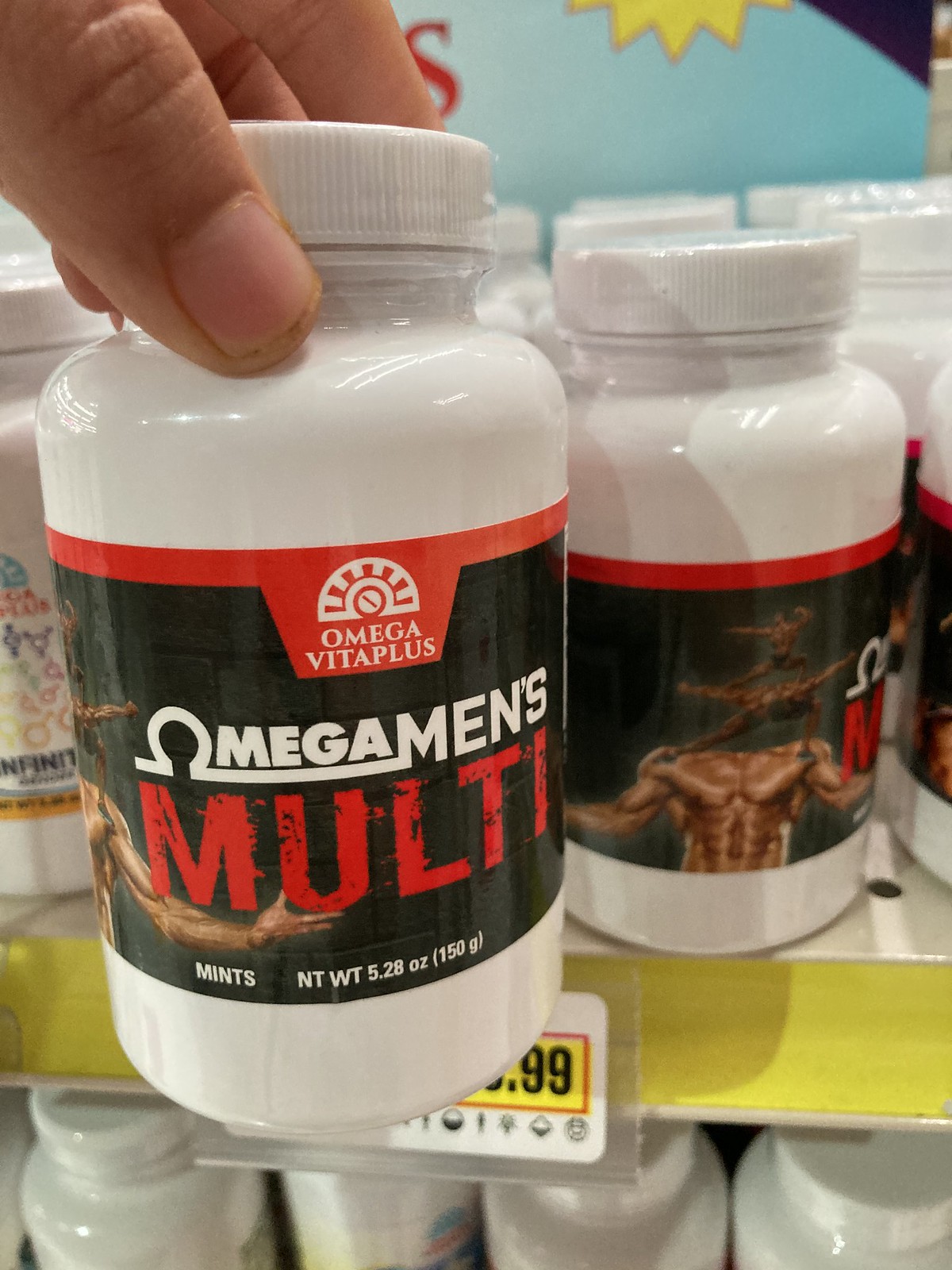In this detailed close-up image, a white pill bottle is prominently featured, held up by someone in what appears to be a supplement store, possibly GNC. The person has taken the item off the shelf to capture a better view of the product. The bottle is partially obscured, revealing only the price ending in "0.99". The label on the bottle reads "Omega Vita Plus Omega Mints Multi Mints net weight 5.28". Surrounding the label are various images depicting muscular men in different bodybuilding poses, adding a dynamic visual element to the label's design. The main image shows a buff, muscular man without a visible head, emphasizing the physique. Additionally, smaller images include another man striking a classic bodybuilder pose and yet another individual demonstrating a similar pose, contributing to an overall theme of strength and fitness.